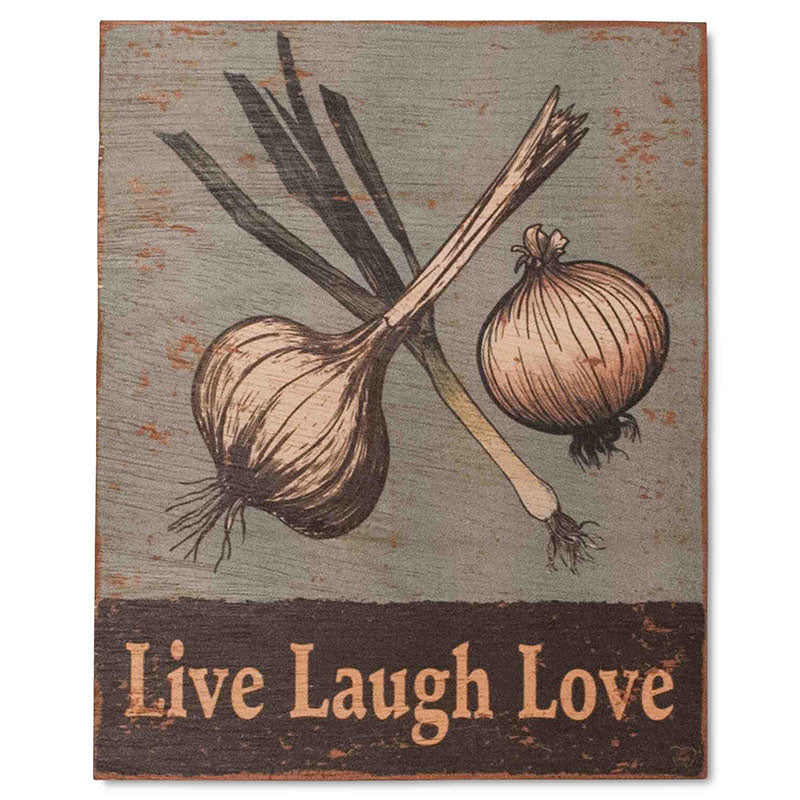This image features a rectangular painting on a light brown, worn-looking board. It depicts a pair of floating onions or possibly a leek, set against a light blue background with visible scratches revealing the brown of the board underneath. The onion on the left is entirely white, the middle vegetable exhibits shades of green, and the right onion has pinkish tints along its edges. The bottom of the board is occupied by a thick black section, taking up about 20% of the canvas. Written in a light, cream color on this black area are the words "Live, Laugh, Love." This vertical artwork, likely intended for kitchen decor, combines a rustic aesthetic with a touch of whimsy.